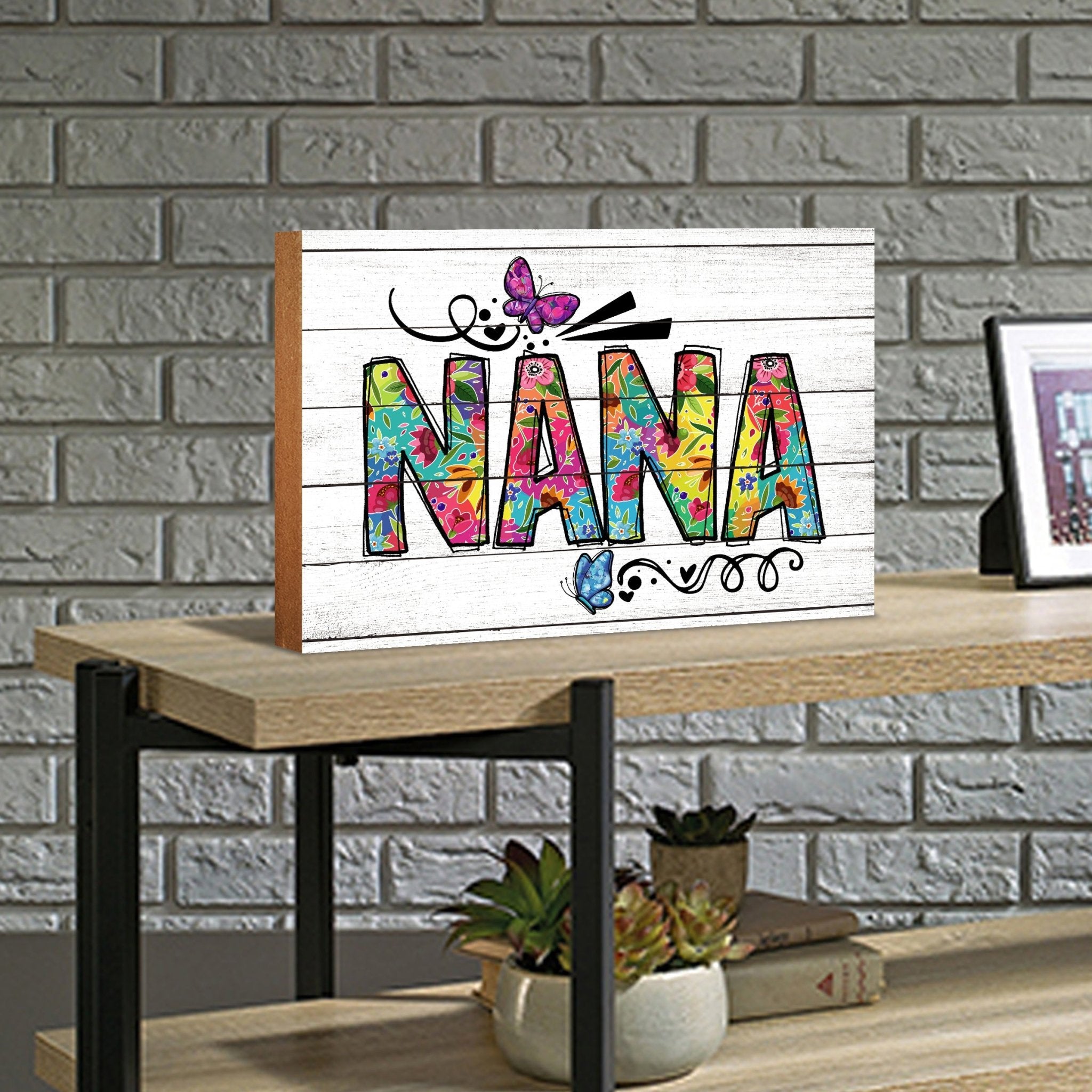The image depicts a digitally created art piece placed on a modern, generic table with two shelves, all set against a plain gray brick wall backdrop. The main focal point is a vibrant, multicolored block text that spells out "Nana" in colors ranging from pink, blue, teal, orange, purple, reds, yellows, and greens, giving the appearance of being adorned with flowers. A white wooden frame, slightly blurred and resembling a superimposed computer image rather than an actual art piece, holds this text. The frame is situated on the right side of the table. Adding to the whimsical design, a purple butterfly is positioned at the top and a blue butterfly at the bottom of the frame. The table itself features black metal arms supporting wood shelves which hold additional decor, including a few stacked books on the lower shelf and some pots with succulents.